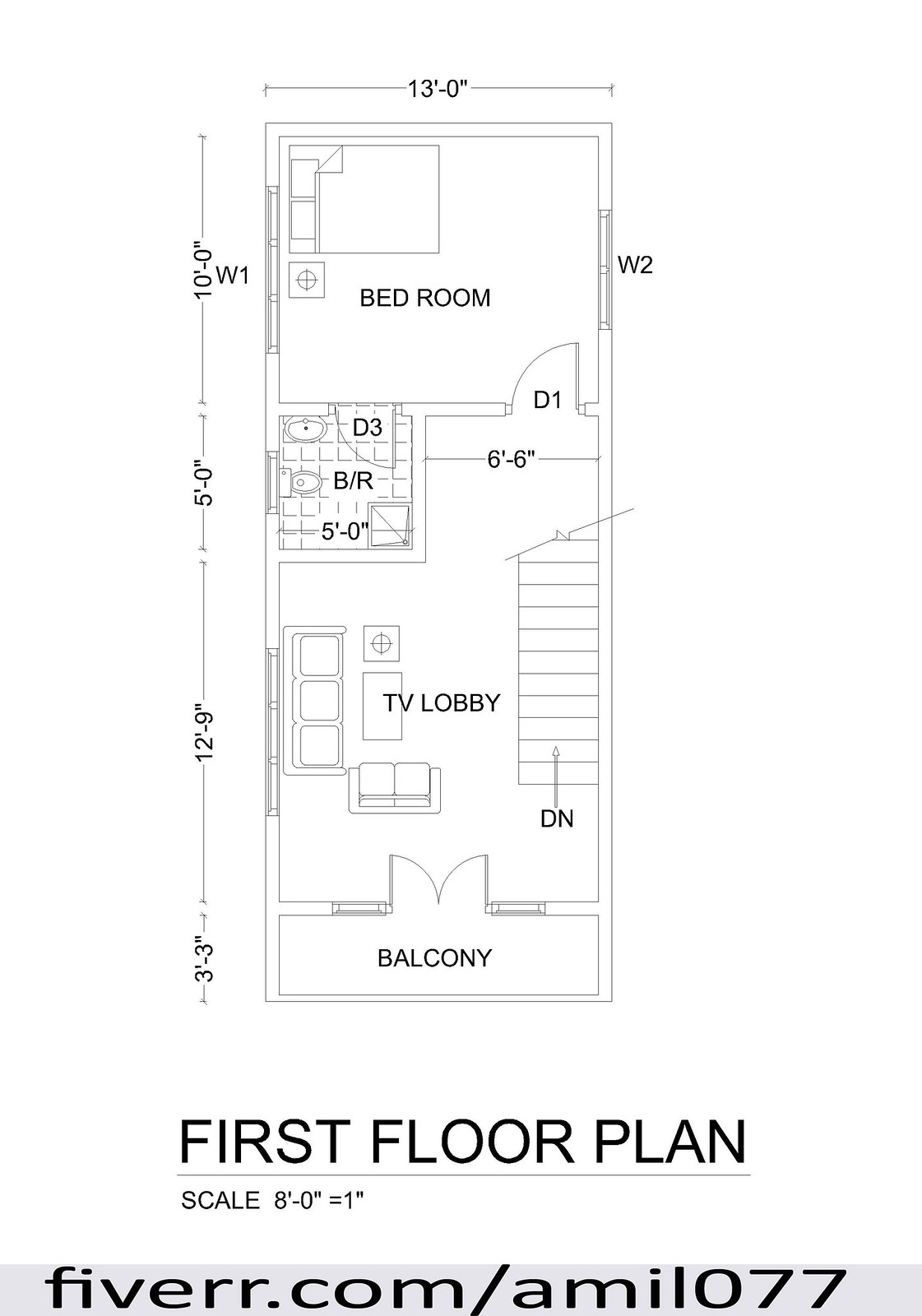"First Floor Plan (Scale: 1 inch = 8 feet): 

The entire first floor is depicted as an extended rectangle. Starting from the top, the first room is the bedroom, measuring 13 feet by 10 feet with two windows situated on opposite walls. The smaller window, labeled W-2, includes a doorway area of 6 feet by 6 inches. Additionally, the bedroom has a doorway that leads into an adjacent bathroom, which measures 5 feet by 5 feet.

Proceeding down from the bedroom, the next room labeled as the 'TV Lobby' features a layout with a couch, chair, and coffee table. The dimensions for the TV Lobby are 12 feet 9 inches long by 13 feet wide. This room extends to a balcony that is 3 feet 3 inches deep and 13 feet wide, providing outdoor access.

The TV Lobby also contains a set of stairs ascending to a presumed second floor. A link at the bottom of the diagram directs to fiverr.com/AMIL077."